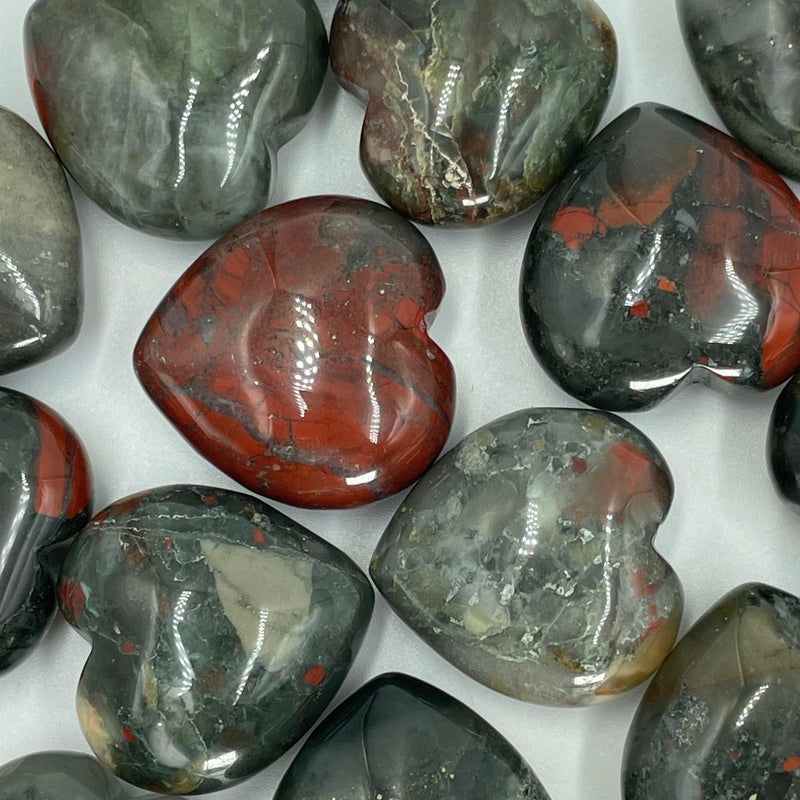The image features a scattered arrangement of heart-shaped stones on a grayish-white background. Each stone boasts a polished and shiny surface, showcasing a variety of intricate patterns and colors. At the top, a prominently shiny heart-shaped rock displays a mix of red, gray, green, and white spots. Directly below, another stone is predominantly red with black lines and white spots running down the middle. Adjacent to these stones is a heart that is green with red spots and pale green or cream splotches accompanied by white dots. Further down, a partially visible dark gray-green heart can be seen. To its right, a partially transparent stone reveals an interior blend of greens, encased in a gray outer layer, highlighted by white spots. Above this is a striking black stone with red streaks and white spots, while next to it lies a stone with browns and greens, also adorned with white spots. Just above and to the right, a sliver of a gray and green heart is visible, with another partially seen black stone below, marked by streaks of color. The stones are not arranged in any particular pattern and have a few cut-off edges, adding to the casual scattered look of the image.